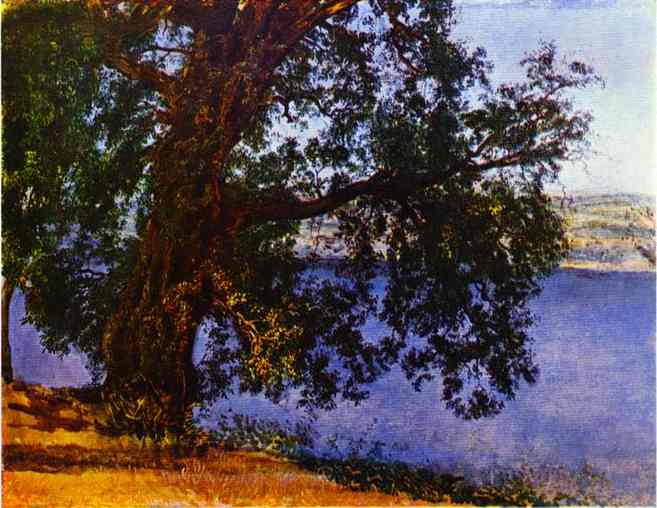This wide rectangular painting depicts a serene landscape featuring a prominent tree beside a tranquil body of water. In the foreground to the left, there is a light brown and orangey patch of grass and dirt, casting shadows that blend into greener and darker tones towards the edges on the right, suggesting a sunlit day. The tree on the left side boasts a thick, dark brown trunk with large branches extending outward, covered in dense, round, and fluffy green leaves. Through the foliage, one can glimpse the calm, deep bluish-purple lake water, with hues of light blue and white reflecting a clear sky above. The horizon reveals a distant landscape colored in shades of green, yellow, and purple, giving an impression of blurred, unfocused mountains or hills under a light blue sky. The brushstrokes are rough yet masterfully executed, enhancing the painting's textured and dynamic quality.